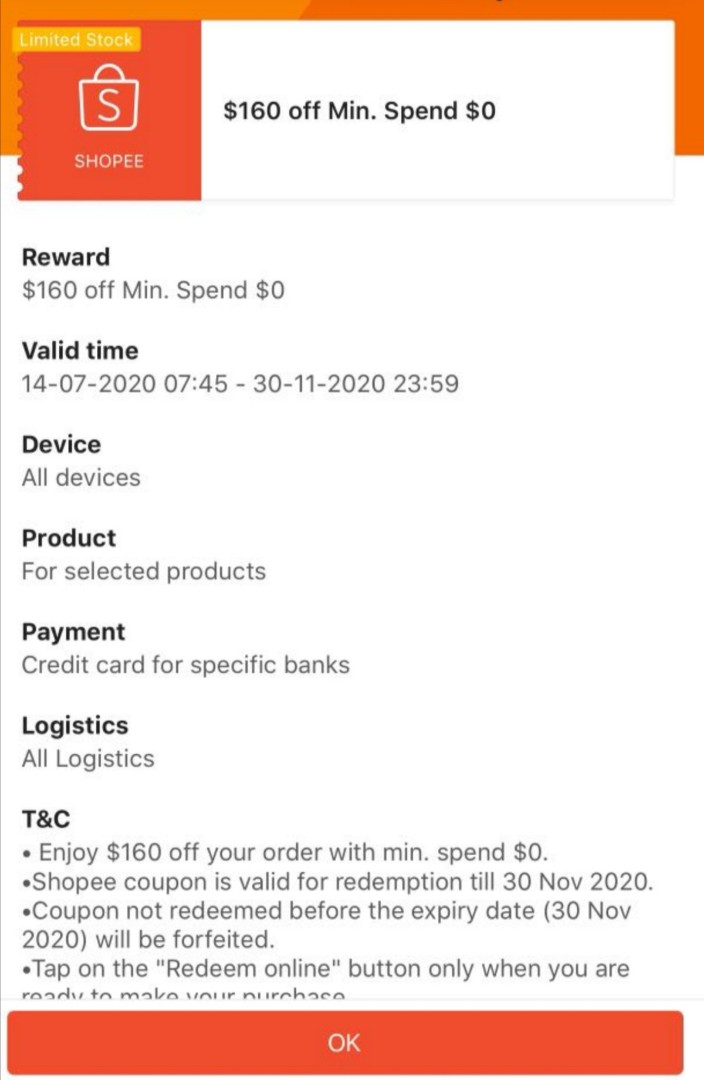This image is a screenshot from the Shopee app, a popular online shopping platform. The central focus is on a promotional coupon offering a significant discount. The coupon provides $160 off with no minimum spend required. Important details about the offer are prominently displayed, including its validity period from July 14, 2020, to November 30, 2020, until 23:59. This promotion is available across all devices but is restricted to selected products and payments made by credit card through specific banks. 

For logistics, all options are supported, ensuring no limitations on delivery choices. Users are reminded in the terms and conditions to tap "Redeem Online" only when ready to finalize their purchase, as the coupon will be forfeited if not used before its expiration. Additionally, there is a clear caution that early redemption could lead to the coupon's loss. 

At the bottom of the screenshot, a red "OK" button is visible, which users can tap to accept and add the coupon to their cart.